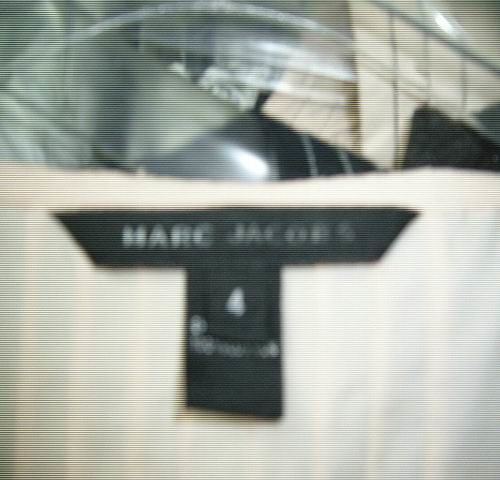The image showcases a Marc Jacobs clothing label, positioned in the typical spot at the top center of the inside back of a garment, such as a T-shirt or jacket. The designer tag is predominantly black with the name "Marc Jacobs" emblazoned in crisp white text in the center. Below the brand label, there's a smaller tag indicating the size "4," although its clarity is compromised due to the overall blurriness of the photograph. Despite the blurred quality, the shape of the number "4" can be discerned. The background hints at the presence of additional clothing items, but they remain out of focus, directing all attention towards the Marc Jacobs label and size tag.